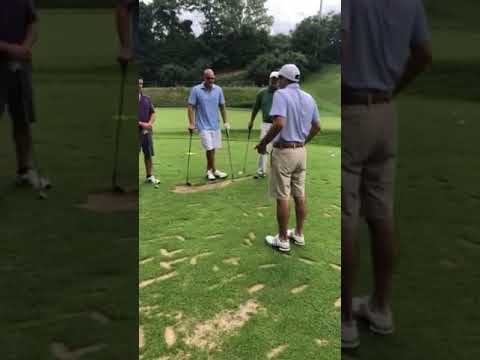The image features four men standing in a row on a golf course during the daytime. The men, who appear to be of African-American, Middle Eastern, or South Asian descent, are all leaning on their golf clubs, waiting to tee off. The golf course appears dry and patchy, suggesting an arid environment. 

On the far left, the first man is dressed in a light blue polo shirt, black knee-length shorts, and white golf shoes. Next to him, the second man is wearing a short-sleeved purple shirt and gray shorts that also go to his knees, with white shoes. The third man, positioned to the right of the second, has a lavender shirt with white shorts and holds two golf clubs, one in each hand. The man on the right end of the group is wearing a green short-sleeved shirt, a white hat, white khaki pants, and white shoes; he is also leaning on a single golf club.

The image has been segmented into three sections: left, center, and right. The left and right sections are zoomed-in versions of the two pairs of men flanking each side. Additionally, there's a hint of another person off-frame towards the back, evidenced by a white shoe and golf club visible in the lower right-hand corner of the image.